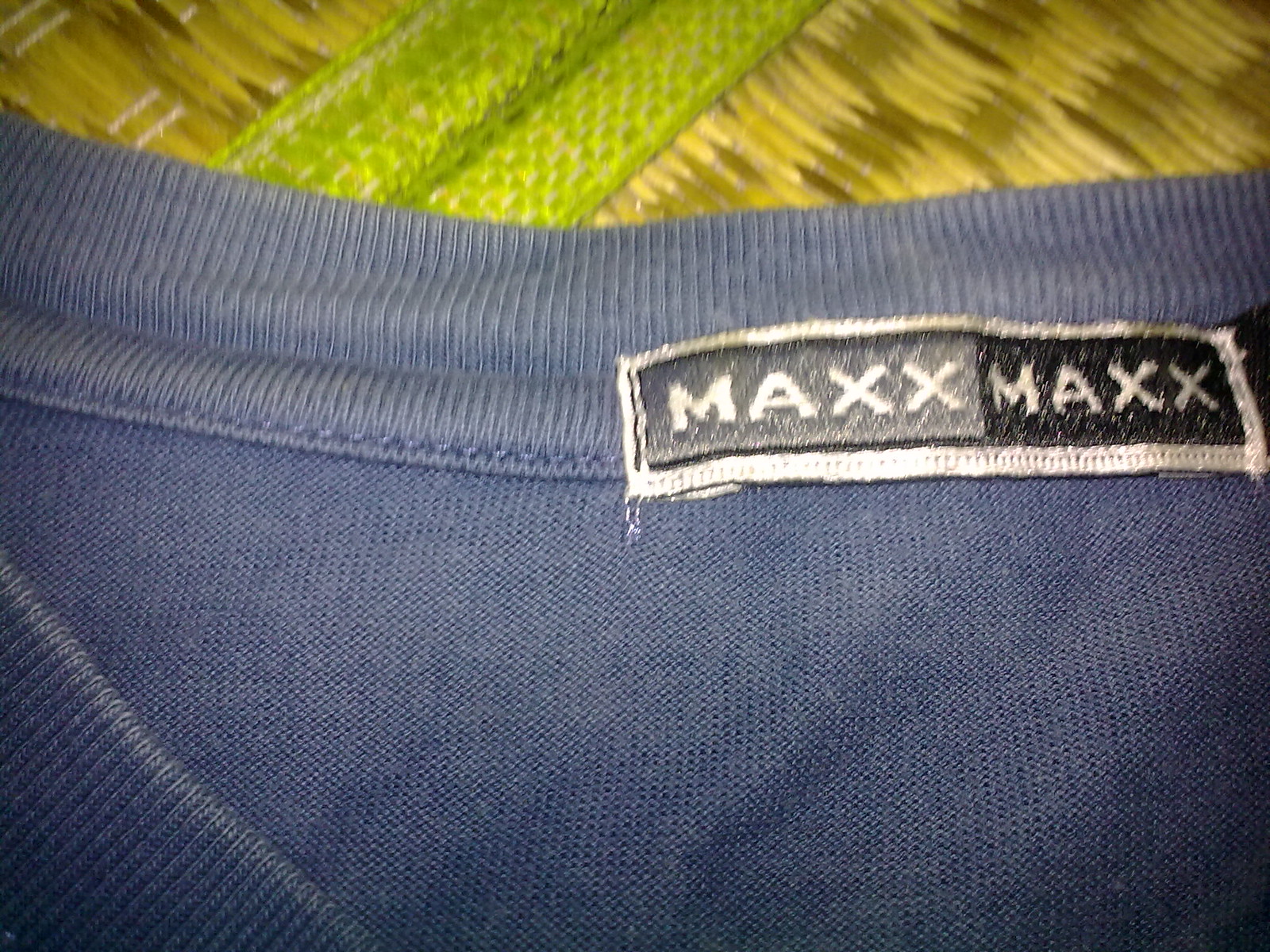The image showcases a light blue, possibly cerulean blue, shirt focused primarily on its tag, which reads "Max Max". The shirt appears to be quite old, characterized by numerous creases and a lack of ironing. Though details of the shirt's complete design are obscured, it seems to feature a V-neck. The tag itself is silver, with black and grey shadowing, providing a stark contrast to the fabric. The shirt is laid on a fibrous table or a roll-down eating surface, adding to the casual and somewhat unkempt presentation of the photograph. The overall setting and style of the image lack professional quality.